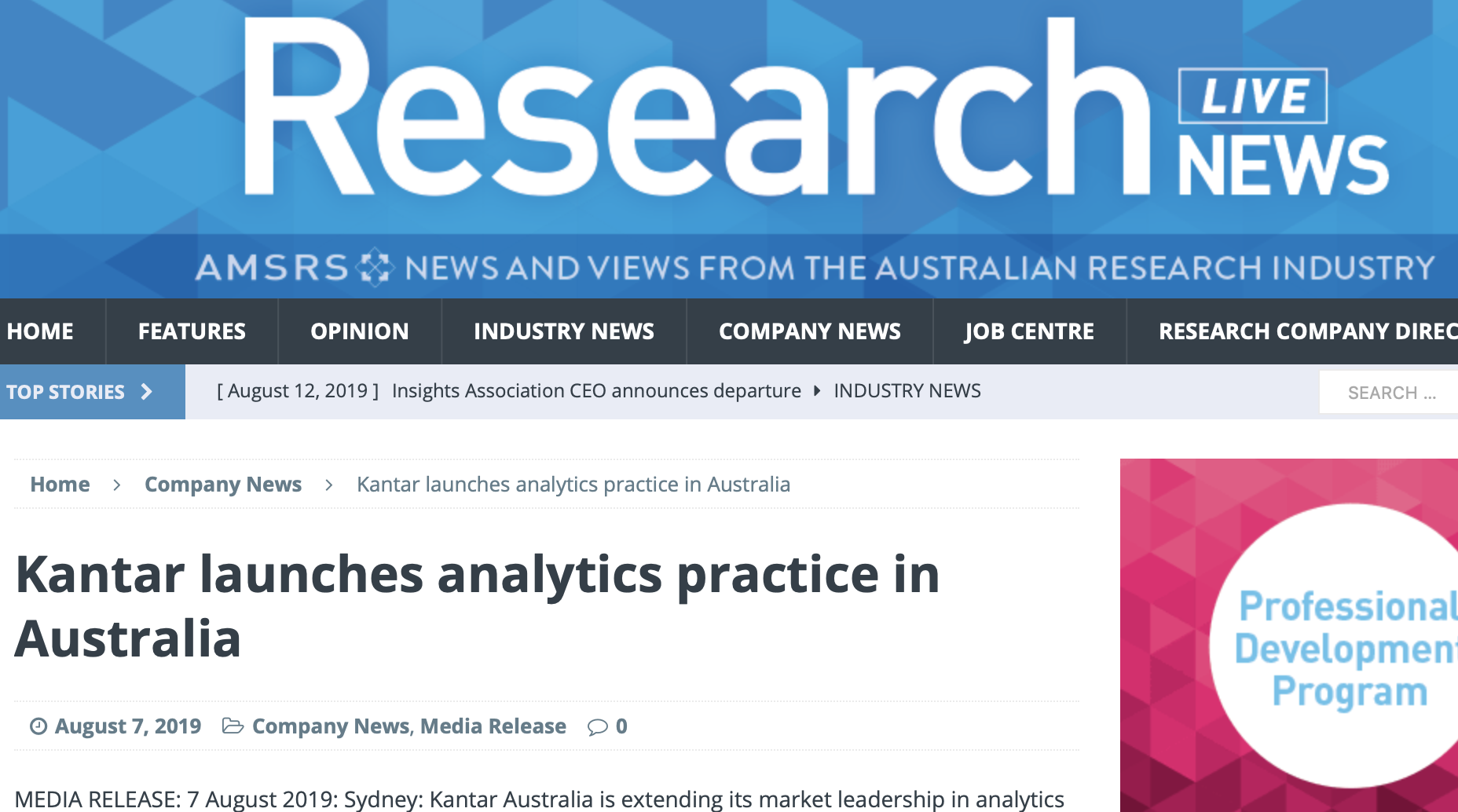The image showcases a detailed screenshot of a computer monitor displaying a research-focused live news website. The top banner prominently reads "Research Live News," with the sub-heading "AMSRS: News and Views from the Australian Research Industry."

Navigational tabs below the banner include "Home," "Features," "Opinion," "Industry News," "Company News," "Job Center," and "Research Company Directory." Beneath these tabs, the "Top Stories" section highlights an article dated August 12th, 2019, with the headline: "Insights Association CEO Announces Departure." To its right, there's a right-facing arrow, followed by an "Industry News" label and a search box.

Further down, there are additional navigation tabs labeled "Home" and "Company News" featuring the caption "Kantar Launches Analytics Practice in Australia." The main article headline "Kantar Launches Analytics Practice in Australia" is accompanied by the date August 7th, 2019, along with icons indicating time and category (Company News, Media Release) with an information bubble showing the number zero. The article starts with "Media Release, August 7th, 2019, Sydney: Kantar Australia is extending its market leadership and analytics."

To the right of the article snippet, there's an advertisement promoting a professional development program.